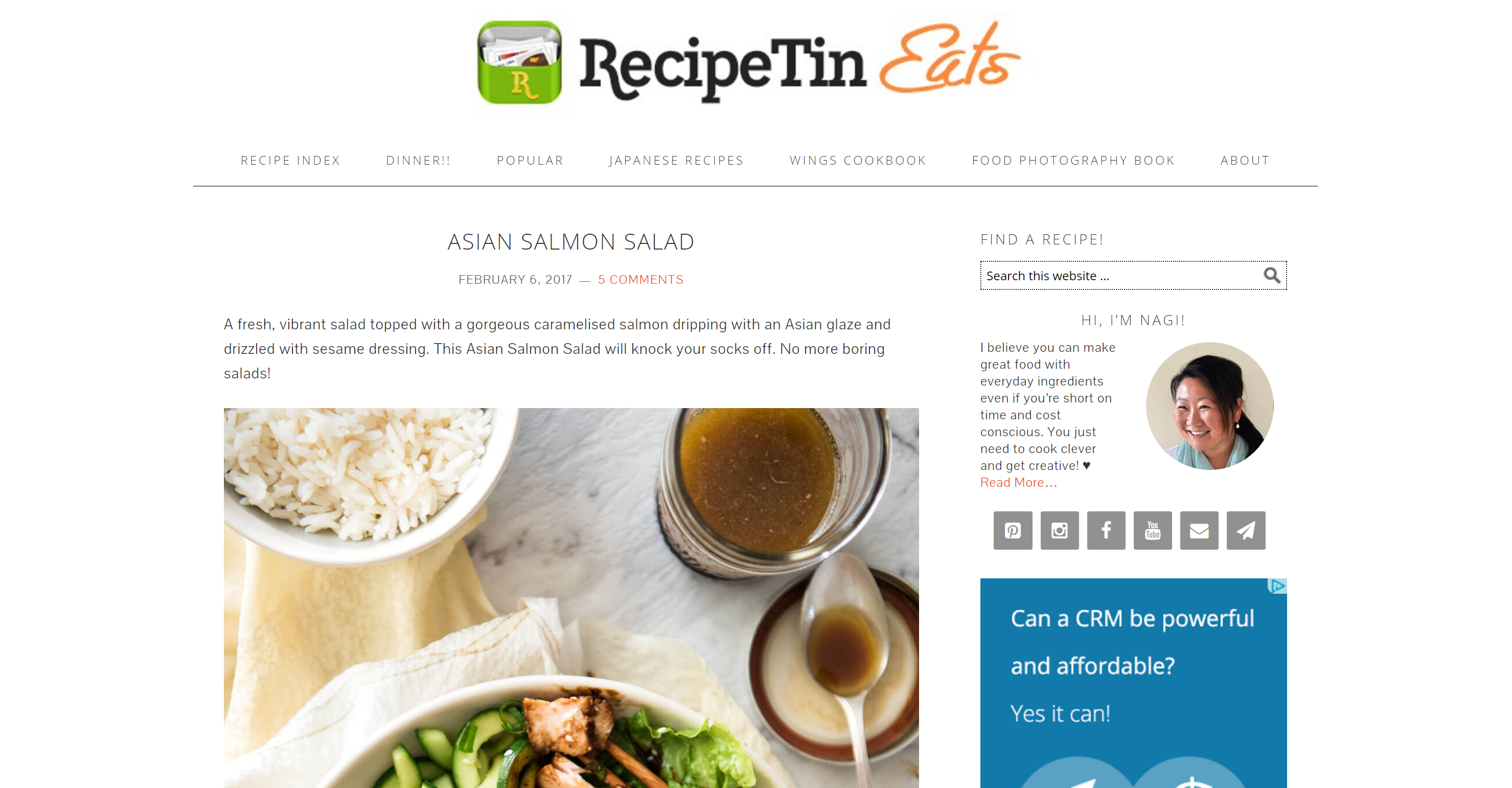The image displays a screenshot of the "Recipe Tin Eats" website. At the top of the page, the logo is prominently featured, consisting of a small green tin with an 'R' on the front, filled with food items. The website's name, "Recipe Tin," is written in bold black letters while "Eats" is highlighted in orange. 

Below the header, there is a navigation bar with grey tabs offering quick access to various sections like Recipe Index, Dinner, Popular, Japanese Recipes, Wings Cookbook, Food Photography Book, and About. 

The main content area showcases a featured recipe for an Asian Salmon Salad. The image of the dish shows a bowl of rice accompanied by various vegetables and a separate dish, providing a visual appeal. Accompanying the recipe are five user comments.

To the right side of the page, there is a small profile picture of the website's author, identified as Nag. She appears to be of Asian descent and offers a brief introduction about herself. Above her profile is a search bar to help visitors find specific recipes or topics.

Below Nag's profile are links to popular social media platforms like Instagram, Facebook, and YouTube, enabling users to follow and interact with her on these sites. There's also an option to contact her via email. Lastly, a blue advertisement for a CRM product is positioned in the bottom right corner of the page.